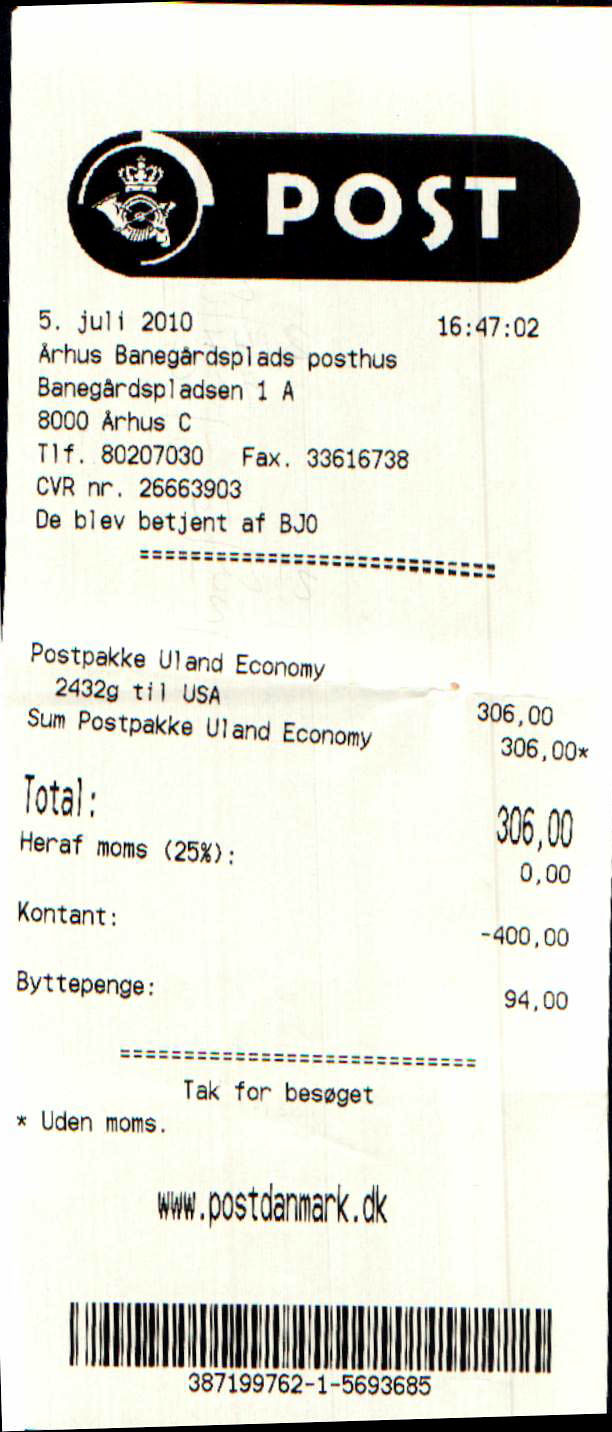The image depicts an aged paper receipt, presumably for a postage service, indicated by the word "POST" prominently displayed at the top within a black circular border featuring white letters. The receipt is dated July 5th, 2010, formatted unusually with "5.JULI 2010" and the time noted as "1647:02" (4:47:02 PM).

The document contains detailed transaction information, including the recipient’s name, "R.S. Bynes Banigal," and other specifics suggesting it's related to international postage, though the exact nation remains unspecified. The receipt lists key details: a recipient number, a fax number, and various other numerical identifiers.

In the center, below a dotted line, the terms "POST," "PACKING," and "ECONOMY" appear alongside "2432 retail USA," hinting that the package weighed around 2,432 grams and was bound for the United States. To the right, "306,00" is likely indicating the cost, possibly in Danish Krone (DKK).

Further down, it notes the total payment and content value with terms like "TOTAL" and "KONTANT." An entry of "–400" suggests a transaction involving 400 units of currency, likely indicating money paid and subsequent change. The ambiguous term "bypins $94" might relate to financial summaries or service fees, albeit in another language.

The bottom of the receipt displays a URL, "www.postdanmark.dk," affirming its connection to Danish postal services, and a barcode, likely a receipt ID for tracking or reference purposes.